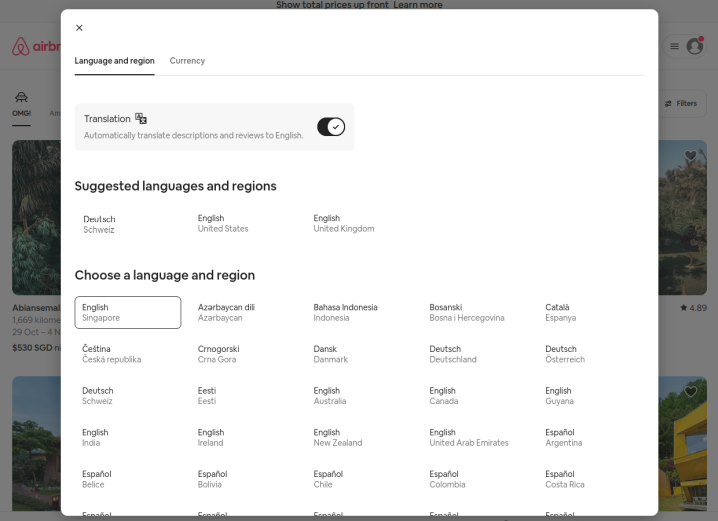**Caption:**

The image features a pop-up interface on a white background. In the upper left corner, "Language and Region" is written in black text and underlined. To the right of this, "Currency" appears in light gray text. Below, the section titled "Translation" states, "Automatically translate descriptions and reviews to English," with a toggle button next to it that is switched on.

Underneath this text, another section in bold black text reads "Suggested Languages and Regions" with options listed from left to right: Dutch, English for United States, and English for the United Kingdom. Further down, another bold black text header states "Choose a Language and Region," followed by a box highlighting "English Singapore." 

The options listed from left to right are: Singapore, Azerbaijan, Indonesia, Bosnia, España. The second row consists of: Čeština (Czech Republic), Snagorë, Denmark, Deutsch (German), Dutch. The third row contains: Dutch, Eesti (Estonian), English Australia, English Canada, English Guyana. Finally, the fourth row includes: English India, English Ireland, English New Zealand, English United Arab Emirates, and Español Argentina.